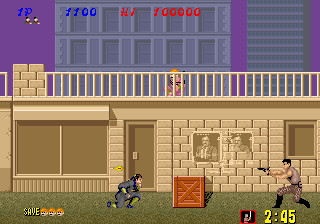In this screenshot from a video game, vibrant yellow text reading "Save" appears in the bottom left corner, accompanied by three face icons. To the right side of the image, a lush patch of green grass contrasts with the action unfolding center-frame. Another set of yellow text displays the number "245". 

The focal point showcases a character actively shooting towards the left while a wooden crate rests nearby. Adjacent to this crate, another character is crouched defensively. They both are positioned in front of a stately stone building featuring detailed brick walls, doors, and windows. Above them, a balcony area is visible, supporting yet another character. The serene, purple sky serves as a backdrop, juxtaposed against the building's additional grey floors. The scene combines dynamic action with a richly detailed environment, seamlessly blending character interaction within a meticulously crafted setting.